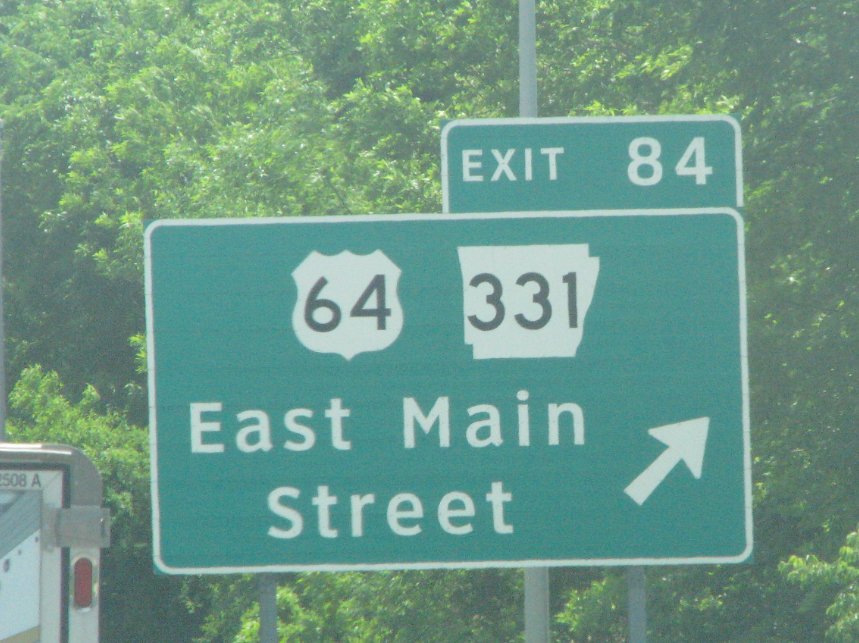This color photograph, taken outdoors on a bright, sunny day, has a slightly hazy and unfocused appearance. The background is filled with leafy trees, casting shadows that add a sense of depth to the image. In the bottom left corner, there is a partial view of a square object featuring a red taillight and the number "508A" at the top. This object appears to be the rear of a vehicle, possibly an emergency vehicle like an ambulance, but not enough is visible to be certain.

The main focus of the photograph is on several large highway signs mounted on galvanized poles. These signs are characteristic green with white reflective edging. At the top is a smaller sign indicating "Exit 84." Below it, a larger sign displays a shield-shaped U.S. Highway 64 marker beside a state road marker labeled "331," though the exact state cannot be identified from the sign's shape. The bottom portion of the sign directs drivers to "East Main Street" with an arrow pointing right, indicating that this is an exit off to the right.